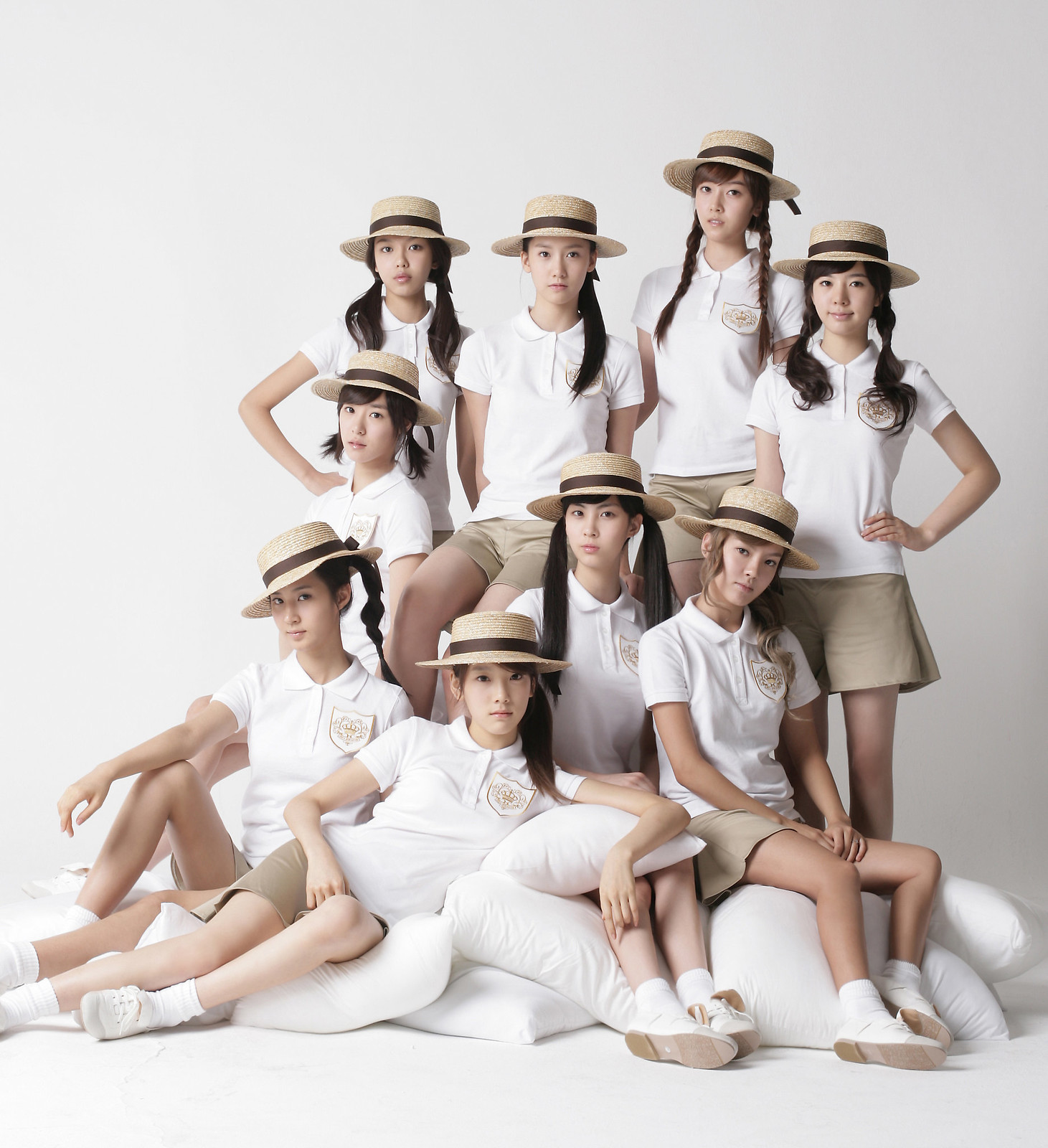This is a detailed photograph of nine young girls posing together in what appears to be a coordinated photo shoot. They are all dressed in private school uniforms, comprising white short-sleeved polo shirts featuring a small brown emblem on the left breast. The uniform also includes brown skorts (shorts resembling skirts), white socks, and white shoes. Each girl wears a light brown straw hat with a dark brown ribbon. Most of the girls have their hair styled in ponytails or pigtails. The arrangement of the group shows four girls seated on plush white pillows in the front, while the five girls in the back are either standing or sitting on higher surfaces. The background is stark white, emphasizing the uniformity and neat appearance of the ensemble. This scene gives off a photo shoot vibe, suggesting the girls might be part of a band or a similarly coordinated group.